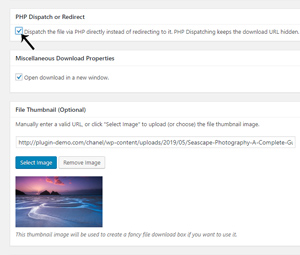This image displays a section of an administrative web page interface for managing file downloads, specifically focusing on PHP dispatch and redirect settings. The interface features a setup where the option to "Dispatch the file via PHP directly, instead of redirecting to it" is enabled. This choice helps keep the download URL concealed. 

In the "Miscellaneous Download Properties" section, the option to "Open downloader in a new window" is turned off. There is also a section titled "File Thumbnail (optional)" where users can either manually enter a valid URL or click the "Select Image" button (which is blue) to upload a file thumbnail image. In this case, a user has entered the address "plugin.demo.com"—potentially a placeholder text. Displayed next to this is a small thumbnail image depicting an outdoor setting with an icy landscape, possibly showing the sun setting.

The page has a white background, with most text in black, and blue highlights such as the aforementioned button. The overall layout and design suggest this is part of a backend web server management tool dealing with PHP-based file handling.